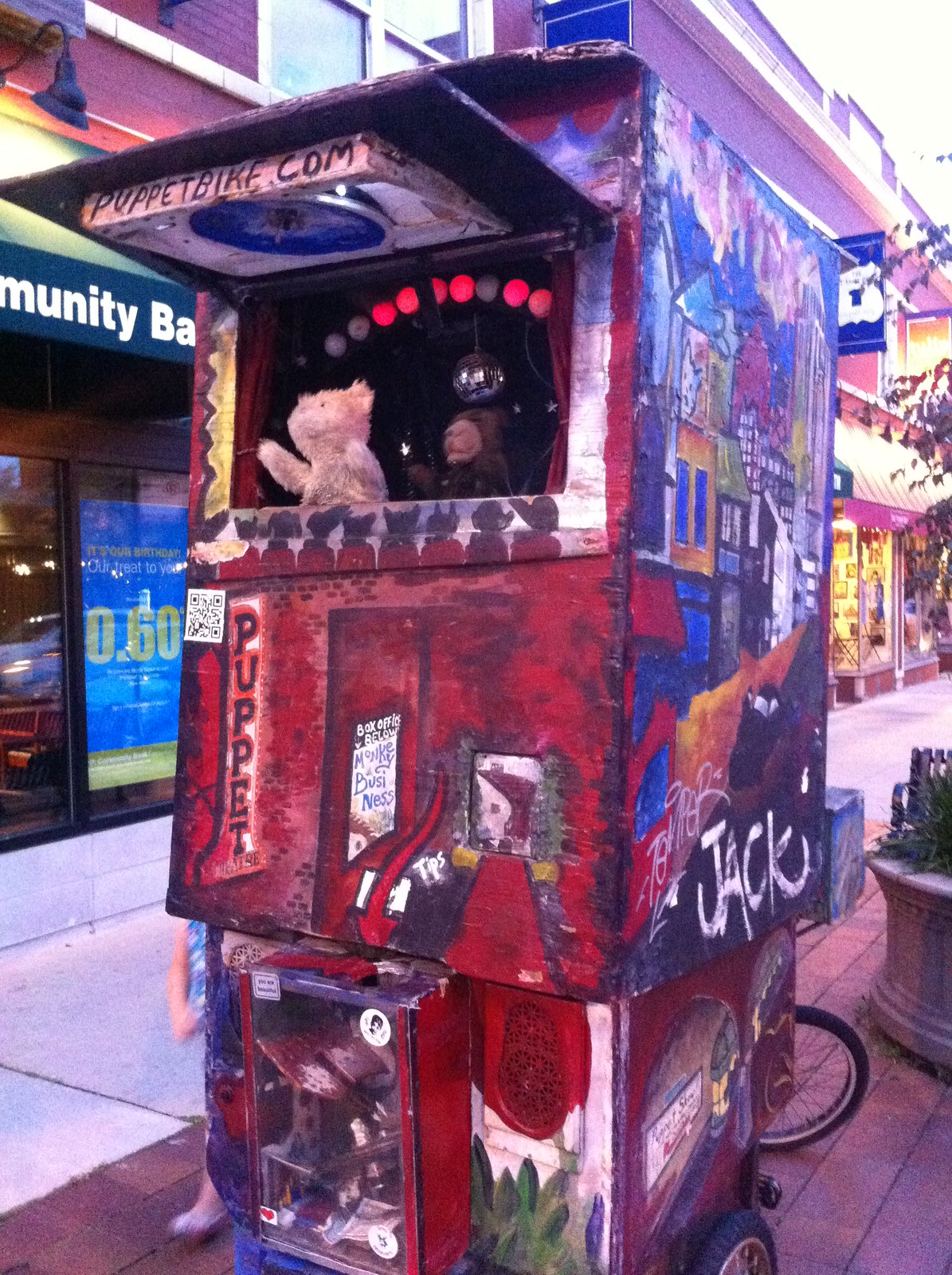In this detailed photographic image, the setting is a bustling city street during the daytime. Central to the image is a vibrant, mobile puppet theater, creatively built behind a bicycle. This artistic kiosk, distinctly marked with a sign that reads "PuppetBike.com," draws immediate attention. The front of the puppet booth is painted red, while the sides are blue, one of which features a charming mural of a town and the word "Jack." Prominently displayed at the booth's front opening is a brown teddy bear, adding to the whimsical allure.

The front of the puppet theater is adorned with the words "puppet" and "bee or monkey business," indicating the playful nature of the performances. A designated tip box is also visible, clearly labeled "tips." Below this, a poster featuring a man's picture adds a personal touch to the setup. 

Additional details include part of a person in a blue shirt and gray pants, with a visible white arm, suggesting activity around the puppet booth. In the background, a series of storefronts and buildings can be seen, including a partly obscured sign for "Community Bank." The ground surface features a brick sidewalk transitioning into a concrete one. The palette of colors in the image consists of gray, tan, blue, dark blue, brown, red, green, yellow, orange, and purple, contributing to the lively downtown ambiance.